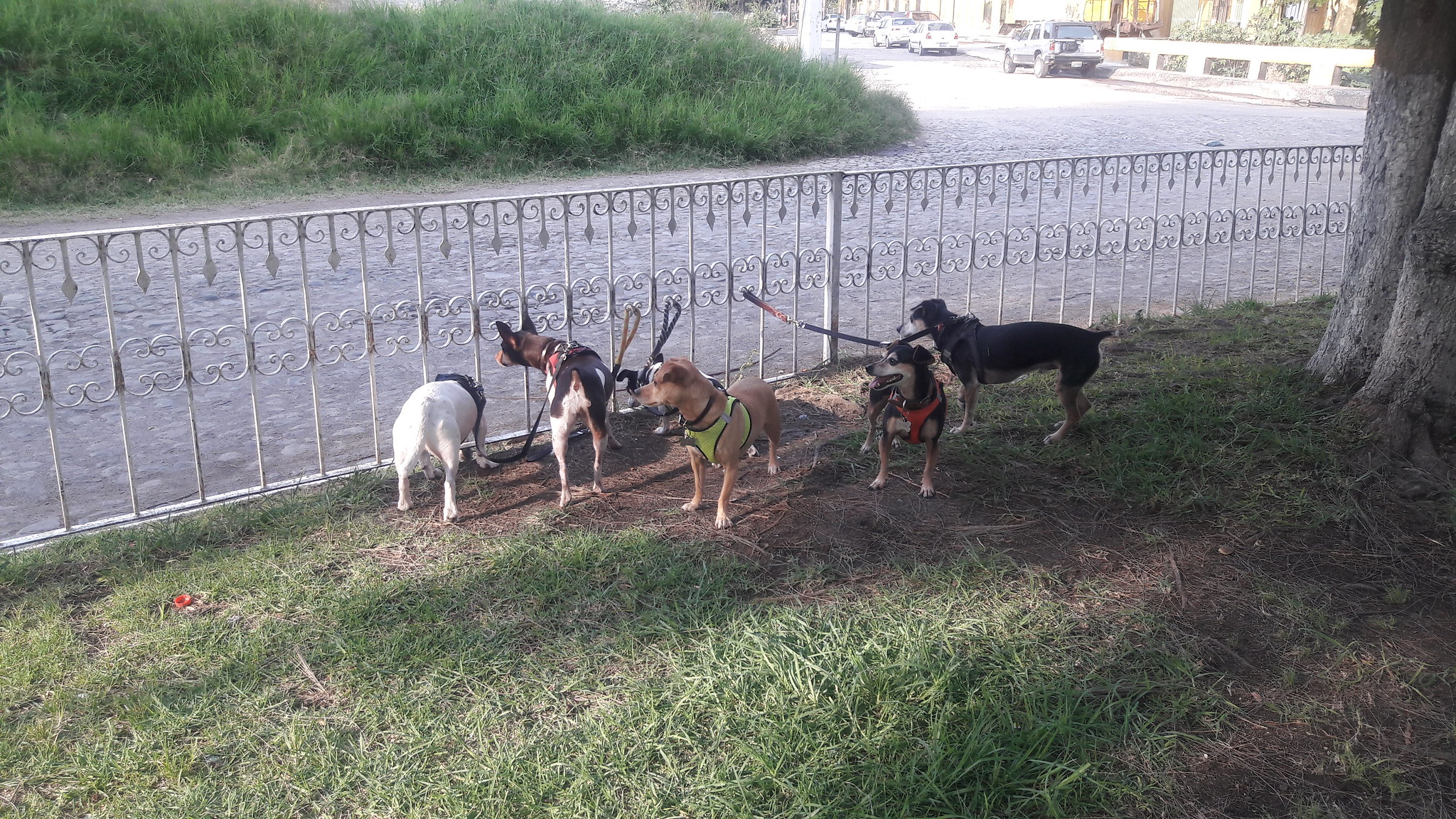In a yard surrounded by a slight rise in greenery and a street lined with parked vehicles against a white partition, five dogs are tied to a white metal fence adorned with light swirl marks and vertical bars. In the foreground, there is a patch of grass, and a tree trunk partially visible on the right side of the image. From left to right, the dogs are positioned as follows: a white dog with a light brown head, a dark brown dog with tall ears and white stripes on its leg, a light brown dog wearing a lime green harness, a black dog with a white face and a red harness, and another black dog with a white face and a black harness. All the dogs are secured to the fence with leashes hooked onto the bars, and appear to be calmly situated in the yard.